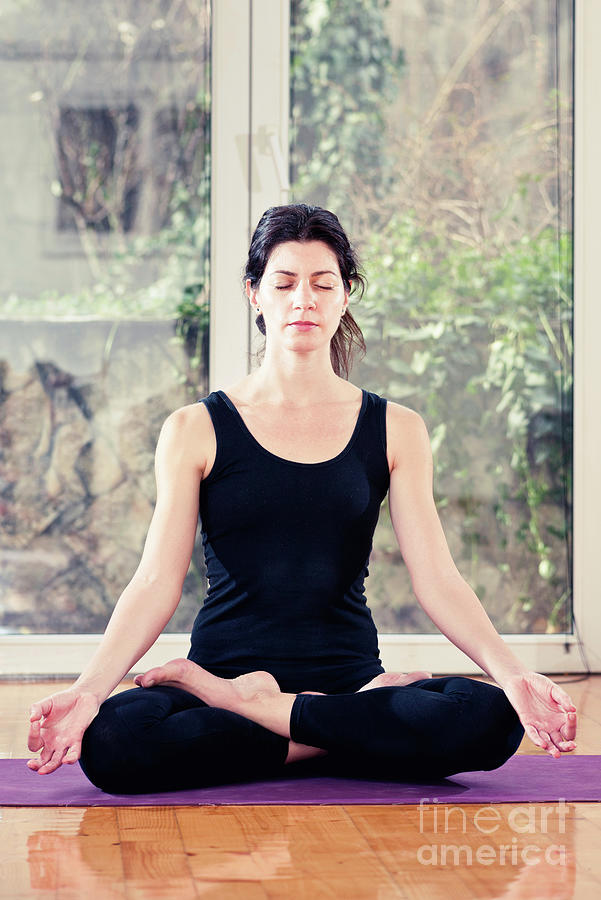The photograph captures a peaceful scene of a woman practicing yoga on a purple mat set on a shiny wooden floor. She is barefoot, wearing a black tank top and black leggings, and her dark brown hair is pulled back in a ponytail. In a classic meditation pose, she sits with her legs crossed, back straight, and eyes closed, radiating tranquility. Her wrists rest on her knees, with her palms facing up and her index fingers and thumbs forming a circle. The backdrop of large, silver-trimmed windows reveals a serene outdoor view of green bushes, nature, and a bit of a rock wall. The space is filled with natural light, enhancing the calm atmosphere. A watermark in the bottom right corner subtly reads "Fine Art America."